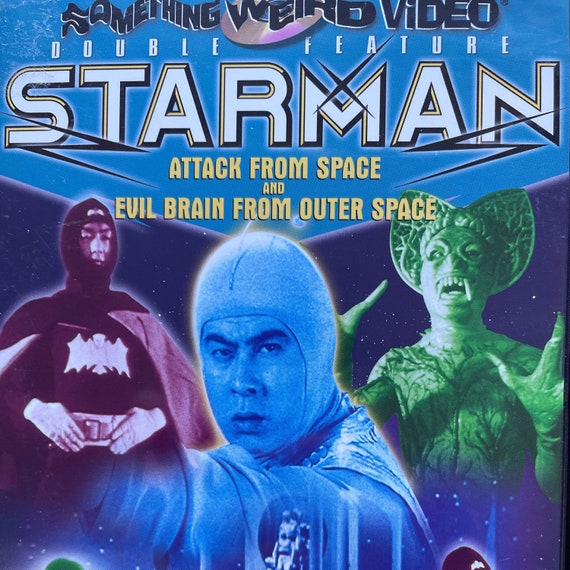This vibrant movie poster is a striking representation of a double feature from "Something Weird Video," prominently showcasing "Starman" alongside "Attack from Space" and "Evil Brain from Outer Space." At the very top, the words "Something Weird Video" are displayed in wavy letters with a CD-ROM or DVD disc behind the word "Weird," followed by "Double Feature Starman" in larger text, with smaller yellow letters announcing "Attack from Space" and "Evil Brain from Outer Space."

The background transitions from light blue at the top to dark blue at the bottom with scattered stars, adding to the cosmic theme. The visual composition includes three main characters at the bottom. On the left, a figure evocative of an Asian version of Batman is dressed in a pale red and black outfit complete with a headdress, cape, belt, and gloves. In the center is a close-up of a man's face marked by intense eyes and thick black eyebrows, adorned with a dark blue and white headdress. On the right, an imposing green lizard-like alien monster brandishes large white teeth and three-clawed gloves, with its arms raised menacingly.

This thoroughly detailed poster serves as a promotional piece for a theater or home video, seamlessly combining the fantastical elements and characters of its featured films.